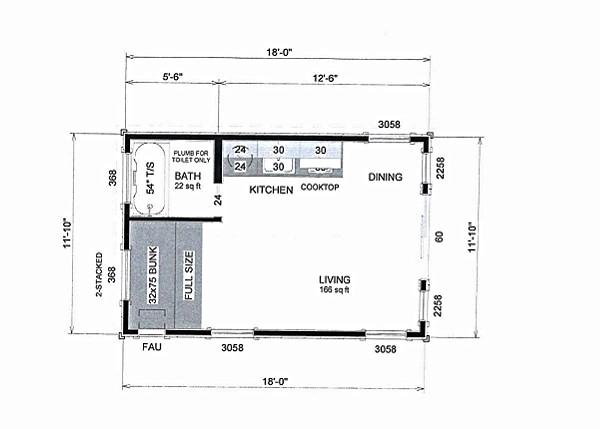This image presents a series of measurements and area specifications in various sections, with text details overlaying a white background. The measurements, which are in black lettering, are highlighted in different shades based on their categories:

1. **Area Specifications**:
    - **Bathroom**: 22 square feet, marked with "54T/S" and indicated to be plumbed for a toilet only.
    - **Living Spaces**: Kitchen, cooktop, dining, and living area collectively cover 166 square feet.

2. **Dimensional Measurements**:
    - **Stacked Measurements**: 11 by 10 inches, two stacked items marked as 358 on one side and 368 on the other.
    - **Bunk Area**: Stated as 27 by 75 inches, labeled as full size.
    - **Higher Area Measurements**: Includes numerical values 18-0, 5-6, 12-6, and 30-58 positioned above the bathroom specifications.
    - **Additional Measurements**: Below the bathroom section, in a white text, measurements such as 24, 30, and 30 are given.
    - **Dark Background Section**: Another set of measurements, 24, 30, with one blank field, followed by details: "kitchen", "cooktop", "dining", "living 166 square feet".
    
3. **Additional Identifiers and Areas**:
    - Notated FAU labeled as 3058.
    - A repetition of the measurement 3058 at another opening, with an adjacent or following record of 18-0.

The image's structured text layout and measurements appear designed to organize spatial layout and utility areas with specific notations and user references for easy interpretation.